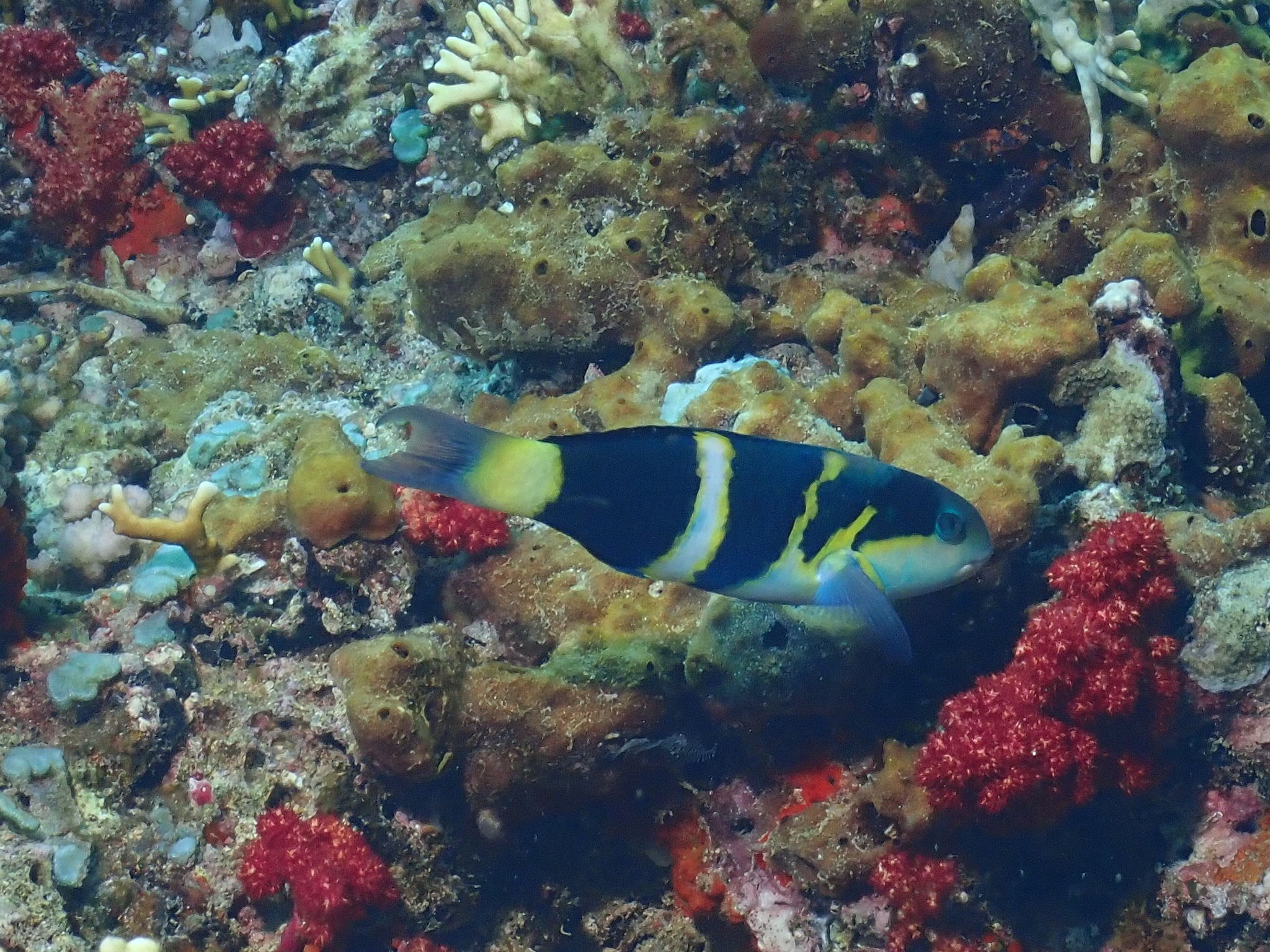In this detailed underwater photograph, a striking, long and narrow fish is prominently featured, swimming from left to right. The fish, shown from its right side, is mainly dark blue or black with distinctive white stripes outlined in yellow. Its dorsal fins are not visible, but its ventral fins are light gray and nearly translucent. The fish has a cream-colored underbelly extending from its mouth down to its middle. The tail is notable for its dark gray color with a yellow base.

The backdrop is an intricate coral reef or an exceptionally elaborate aquarium setting, teeming with diverse marine life. The coral environment features typical beige-green corals interspersed with bright, berry-colored elements, predominantly reds and oranges, creating a colorful tableau. These vivid red globs appear in several locations: the upper left, the middle bottom towards the left, and the bottom right of the image, with additional orange hues extending upwards. Among these vibrant colors are lighter patches of gray, beige, and soft blues, enhancing the visual richness of the scene.